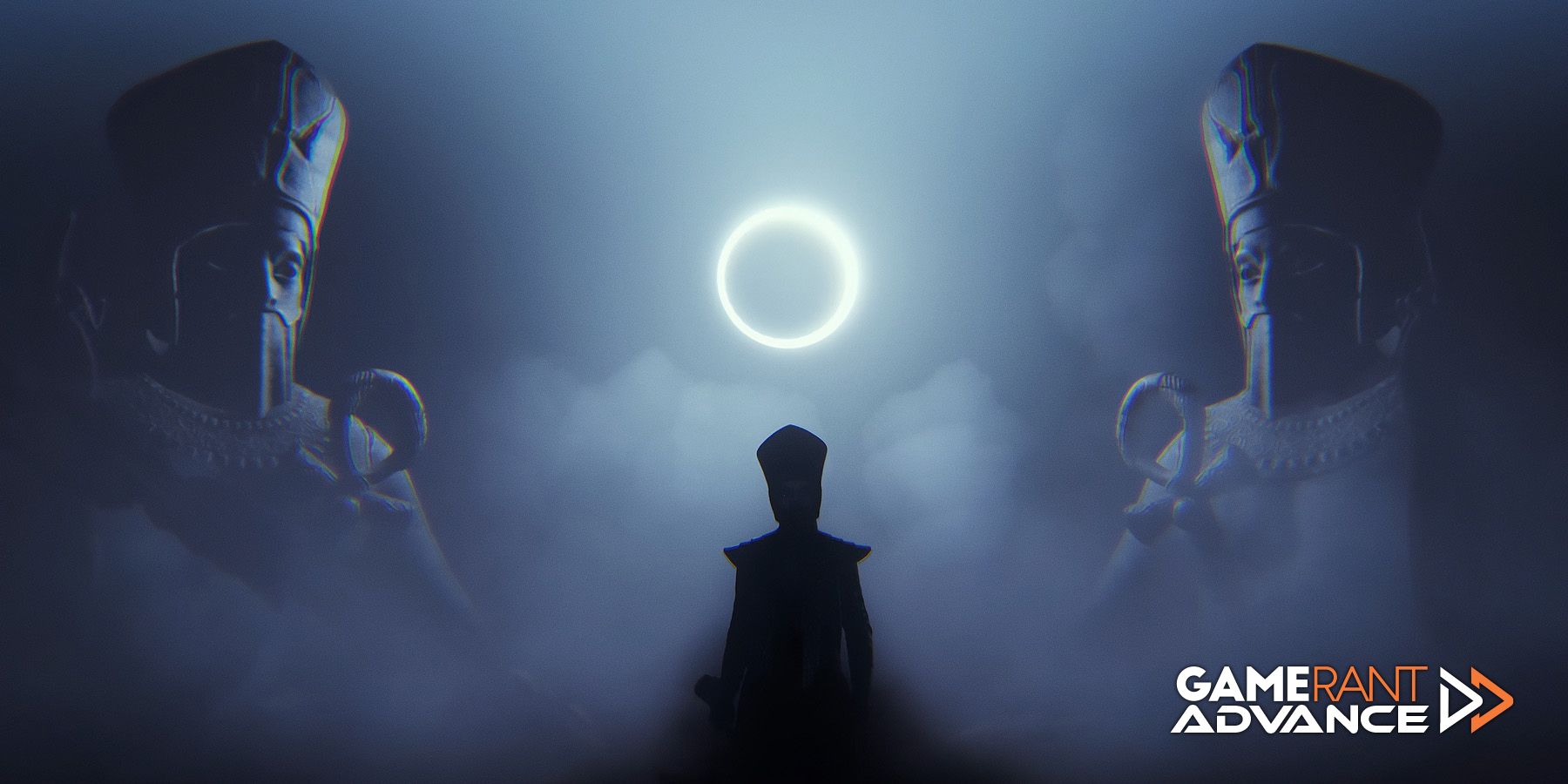The image appears to be a digitally rendered web page featuring detailed computer graphics. In the lower right corner, the logo "GAME" in white uppercase letters and "RANT" in orange uppercase letters is presented prominently. Below this, the word "ADVANCE" is stylized in all caps. Adjacent to the text is a white triangle pointing to the right, layered over an orange triangle pointing in the same direction.

The central focus of the image includes a black silhouette of a person positioned against a backdrop that resembles a solar or lunar eclipse, with a glowing white ring in the center of a cloudy, gray, and dark blue sky. Flanking this silhouette are two stone figures that appear to be of Egyptian origin, each holding a staff topped with an ankh, symbolizing life. The statues, identical to the main figure, wear ornate, religious headwear, further emphasizing a ceremonial or iconic theme.